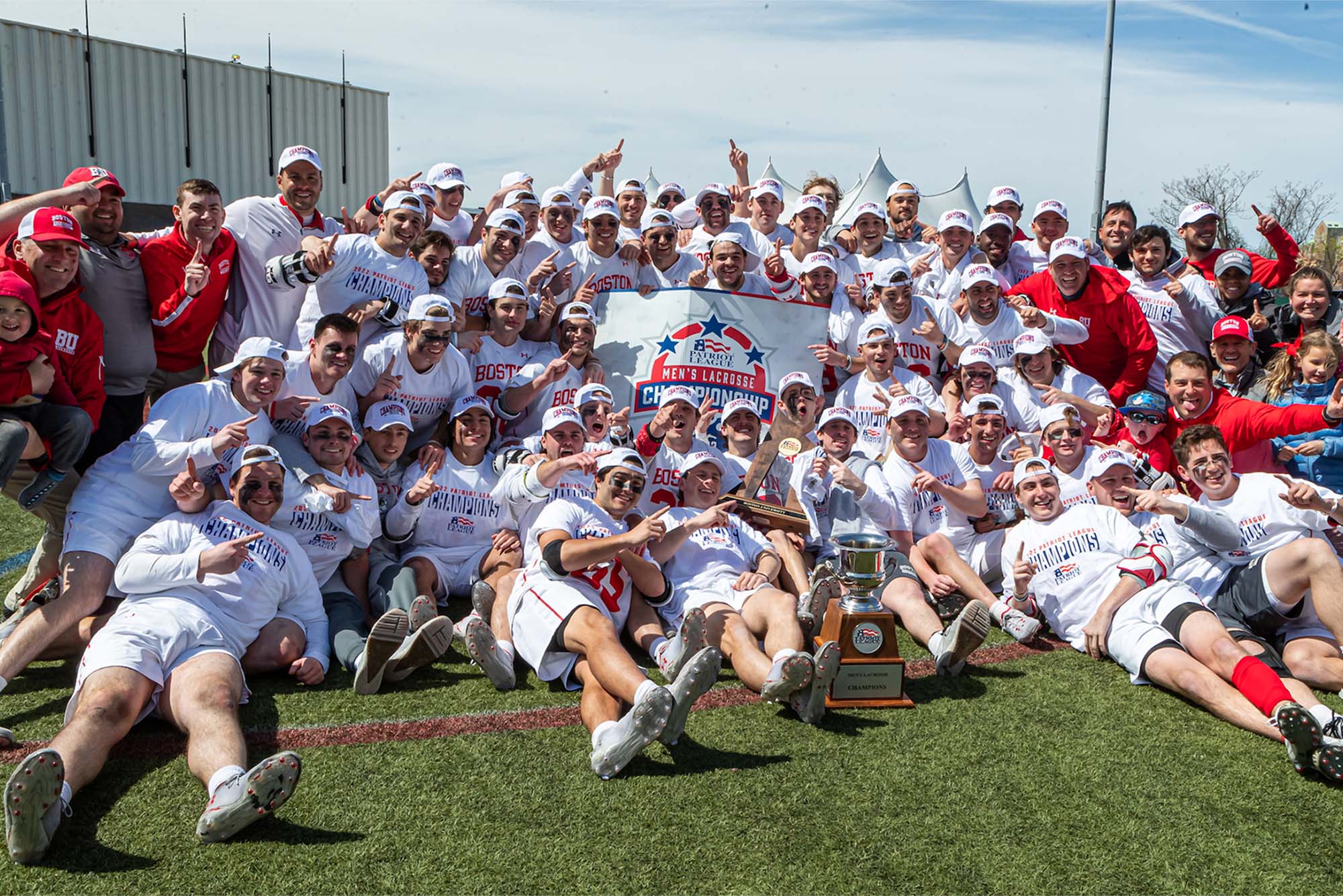The photograph captures a jubilant outdoor celebration of a men’s lacrosse team after winning the Patriot League Men's Lacrosse Championship. The setting is a field with green grass and some brown markings, under a bright daytime sky adorned with white clouds. The majority of the group consists of males, most of whom are adorned in white jerseys, shorts, caps, and sports shoes, while others don red jackets and caps, possibly indicating coaches or staff. The centerpiece of the image is a banner reading "Patriot League Men's Lacrosse Championship," held proudly by some team members. A trophy rests on the ground in front of the team, further emphasizing their victory. Their wide smiles and victory signs, with some team members standing, some sitting, and others lying on the grass, reflect their excitement and happiness. The photograph also features a building or structure in the background, adding depth to the scene. Overall, the image vividly captures the elation and camaraderie of the team in their moment of triumph.